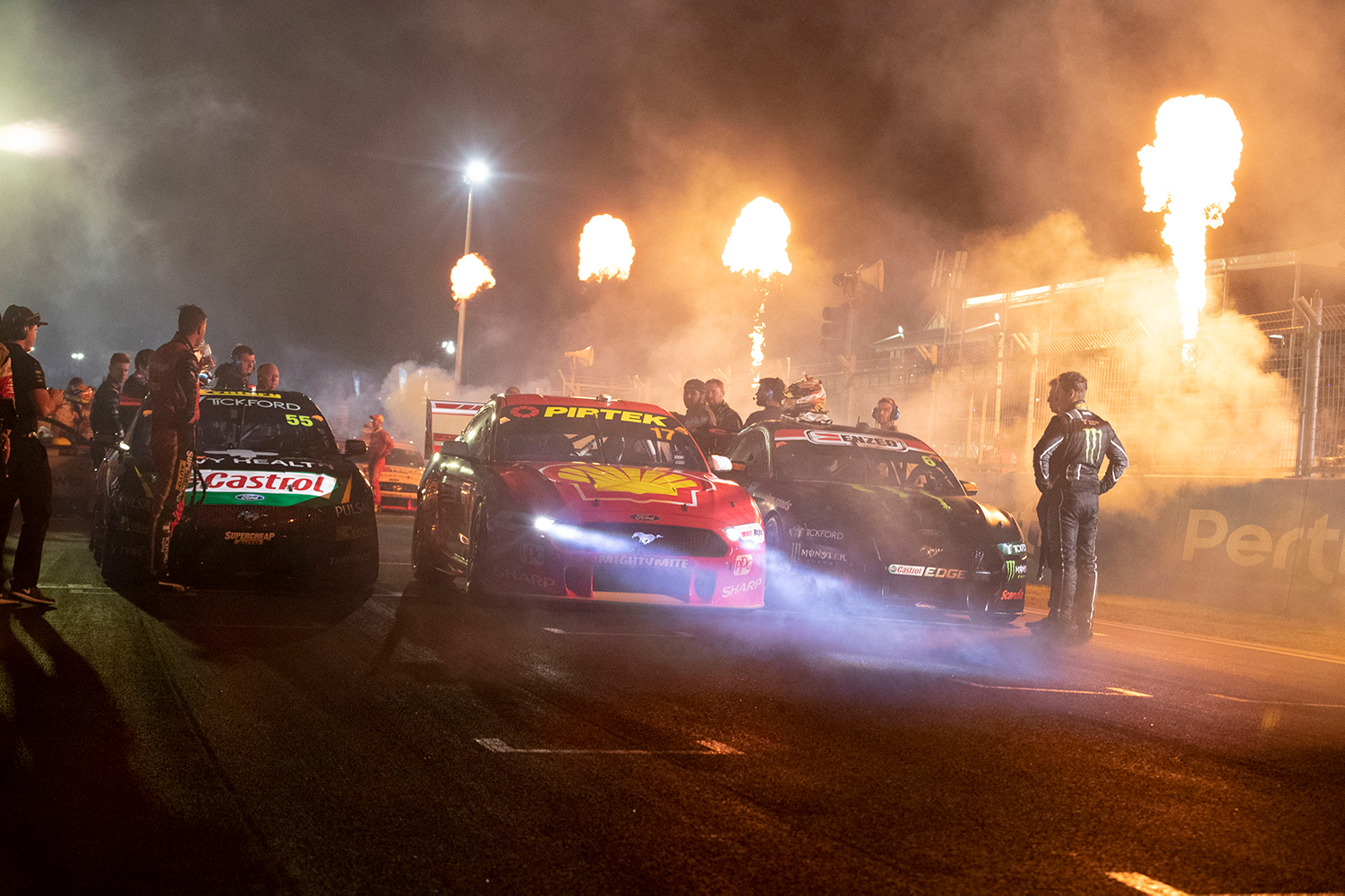In this nighttime image taken at an American racetrack, three distinct race cars are parked on the track, surrounded by a bustling scene of drivers, workers, and racing team members. The black car on the left features a Castrol advertisement and has a distinctive white stripe down the center with red text. The middle car is a striking red with its headlights on and prominently displays a Shell logo on the hood, while the car on the right is also black, resembling a Ford Mustang, with various smaller sponsor stickers, including a notable Monster sponsorship.

Amid the flurry of activity, some individuals are equipped with helmets, while others wear headsets and race jerseys. The atmosphere is charged with excitement as crowds gather around, especially on the left side of the image. Adding to the spectacle, four columns of bright, hot flames—like jets of fire—shoot up in celebratory fashion, casting an intense glow and creating smoke, suggesting pyrotechnic razzmatazz unique to such events. This pre-race moment captures the anticipation and high energy before the cars roar to life on the track.